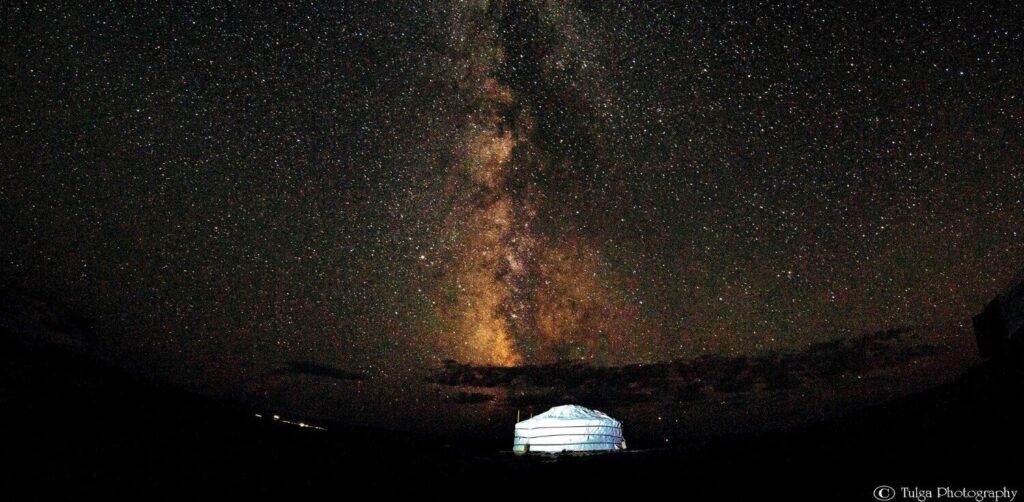In this mesmerizing night sky photograph, 90% of the image is dominated by a breathtaking celestial display free from any city light interference. At the bottom third of the photo, a solid black landscape anchors the scene, featuring a lit, white, domed tent-like structure central to the image. Above this structure, there is a row of dark clouds silhouetted against the starlit sky, adding a mystical touch. The sky itself is a canvas of thousands, if not hundreds of thousands, of white specks representing the stars. A striking Milky Way-like feature stretches up from the horizon, showcasing a radiant display of orangish-pink hues interspersed with subtle greens and purples, resembling a luminous nebula. This stunning composition invites viewers to lay back and marvel at the vastness of the universe, bringing a sense of awe and a reminder of our small place within it. This image, captured by TULGA Photography, combines astrophotography brilliance with a serene earthly element, making it a true visual masterpiece.